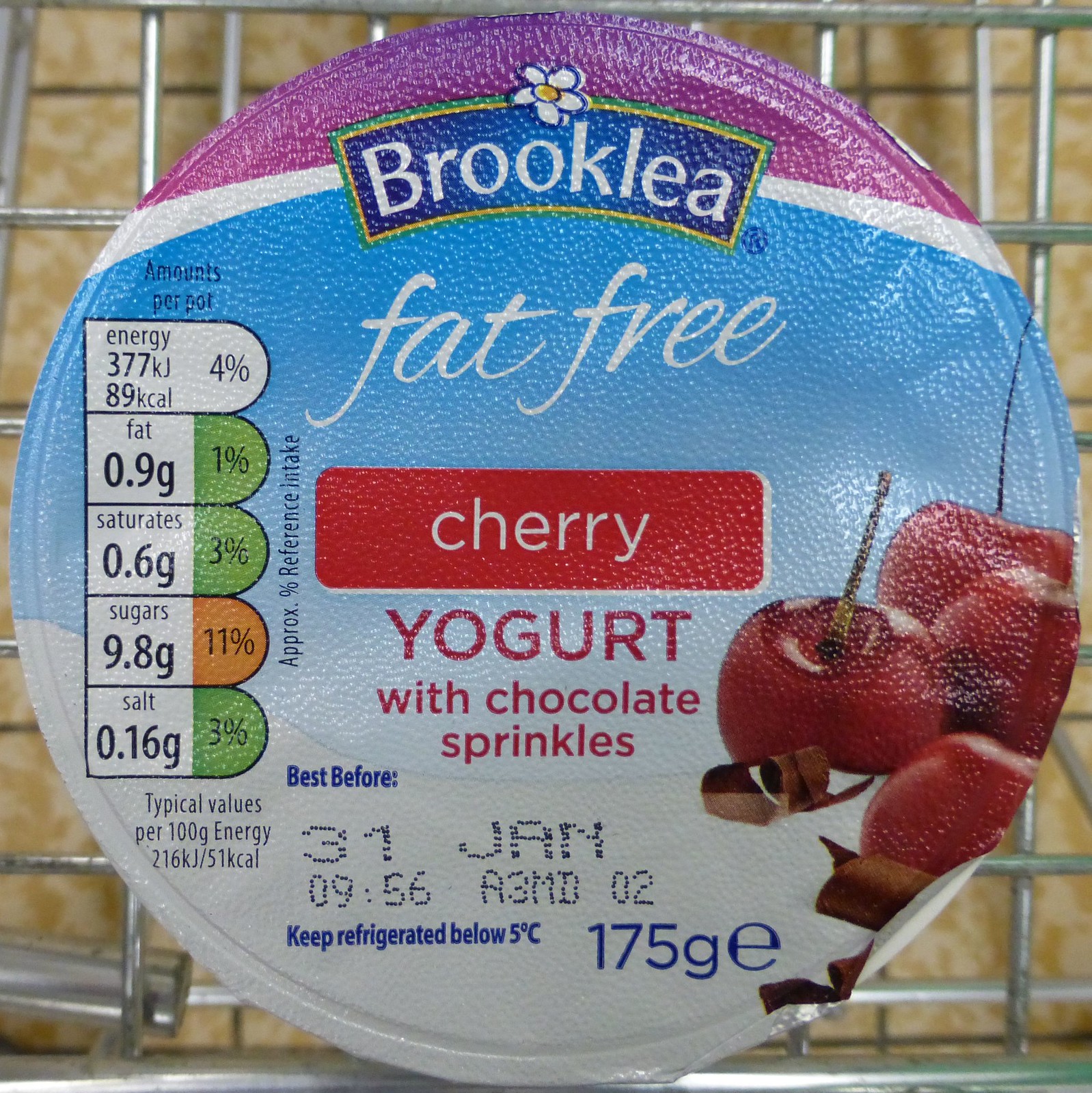This is a close-up photo of a Brooke Lee fat-free yogurt container's lid, likely taken inside a shopping cart, as suggested by the visible metal grates in the background. The lid is predominantly purple at the top with a rounded white stripe transitioning into a blue ombre effect toward the bottom. The top features the brand name "Brooklea" in distinct white font on a blue background, bordered by yellow and green, accompanied by a simple white flower with a yellow center. Beneath the brand name, "fat-free" is elegantly scripted in white, and below that, a red box with white lowercase text indicates the flavor: "cherry." Following this, in capital letters, it states "YOGURT" with the description "with chocolate sprinkles" in lowercase letters.

To the right of the text, there are visually appealing images of four cherries and curved chocolate flakes, highlighting the flavor. On the left side of the lid, the nutritional information is displayed: energy 4%, fat 1% (0.9 grams), saturates 3% (0.6 grams), sugars 11% (9.8 grams), and salt 3% (0.16 grams). The percentages for fat, saturates, and salt are highlighted with green, while sugars are in orange. At the bottom of the lid, there is text noting the best before date ("31 January") and storage instructions ("keep refrigerated below 5 degrees Celsius"), as well as the net weight of 175 grams.